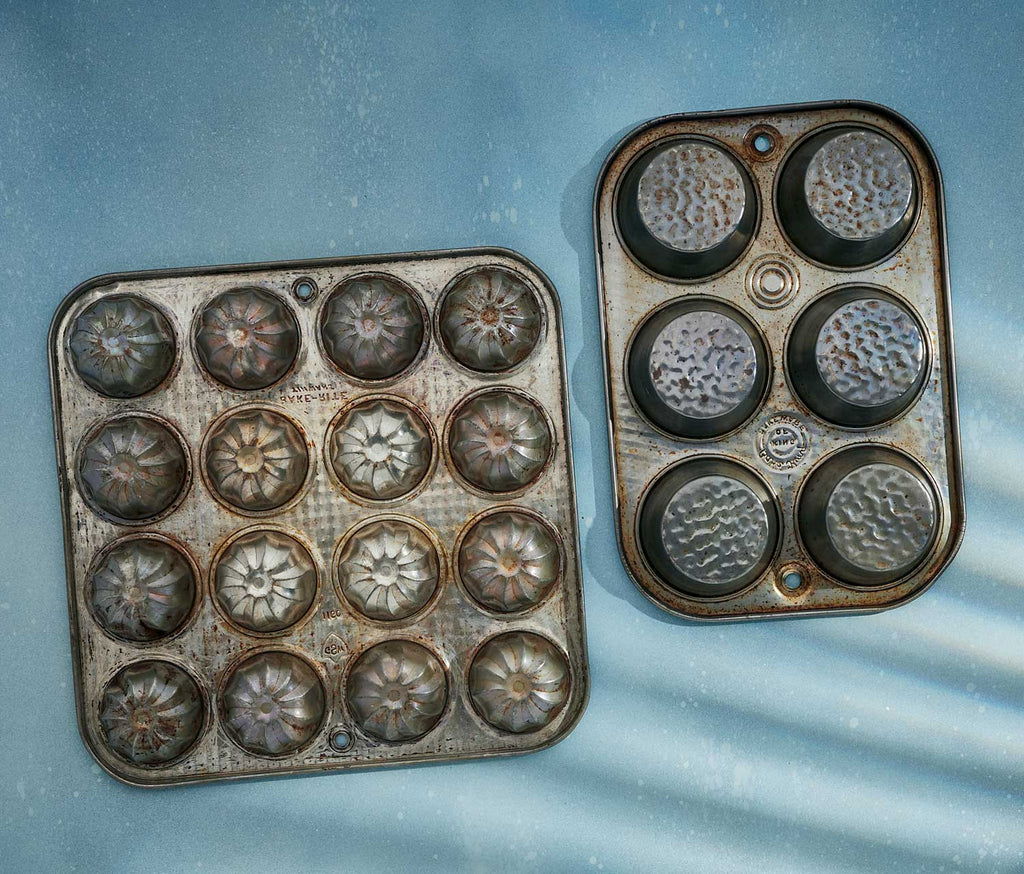The photo features the underside of two old and well-used muffin tins placed on a blue tablecloth. The tin on the left, which can bake 16 small bunt cakes, is arranged in a four-by-four grid and appears somewhat rusted with silver accents showing through its worn surface. The indentations from the molds are clearly visible, suggesting frequent use. The tin on the right, designed for six regular muffins, has a simpler, flatter design and is noticeably smaller in size. It shows significant signs of use, with the bottom almost entirely blackened from grease. Both tins reflect their age and extensive use.